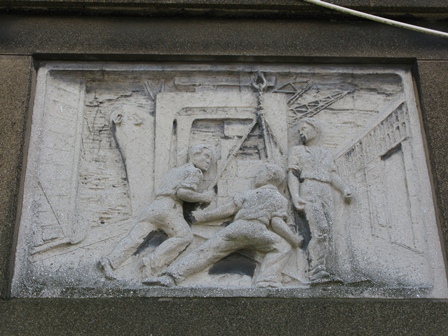The photograph captures a detailed stone carving set within a gray, stone or concrete frame, positioned centrally either inside or outside a building. The scene, rendered in shades of gray and light gray, depicts three male figures engaged in manual labor, with an air of industrious effort. Two men, appearing to face each other, give the impression of either fighting or collaborating intensely, while the third man stands, gazing down at the two, possibly overseeing the activity. The surrounding stone wall features intricate carvings and patterns, which add depth and historical context to the image. The overall ambiance suggests a scene from an old-time setting, evoking a moment of labor or conflict immortalized in stone.